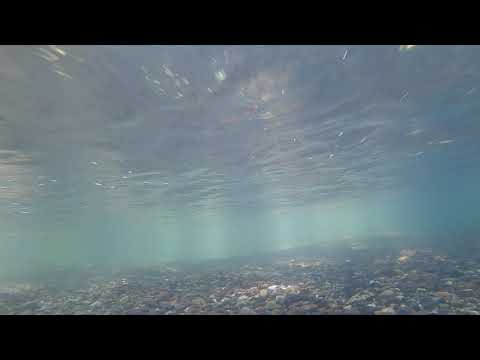The underwater image captures a serene and transparent aquatic landscape, framed by thick black borders at the top and bottom. The water is exceptionally clear, allowing a detailed view of the rocky floor below, littered with a myriad of small rocks, stones, and pebbles. The ground ascends gently to the right, creating a soft incline. The water's surface reflects these earthy, textured elements, giving the image an enchanting, multi-layered appearance. Sunlight penetrates through the water, casting bright rays that create a naturally lit scene and highlight the variety of colors in the water, ranging from dark blue and green to whites and browns. The image, taken during daylight, exhibits no human presence, animals, words, or numbers, emphasizing the natural beauty of this tranquil underwater environment.